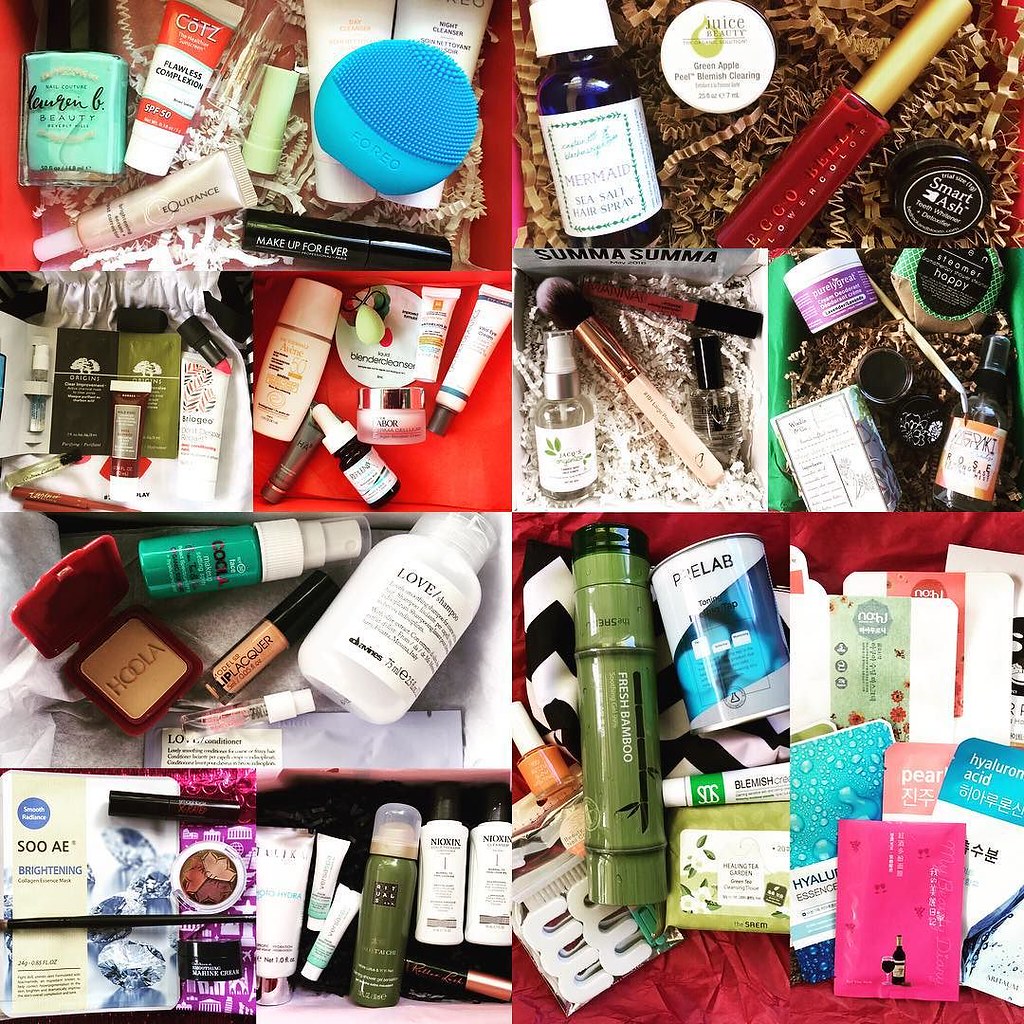This photograph showcases an assortment of makeup products neatly organized, resembling either a drawer or a packaged set ideal for travel. On the top right, there's a distinct long red item resembling a popsicle, with a thick brown or beige handle. This red object appears soft and features yellow buttons. Surrounding these items, brown twirly packaging material is visible, providing a textural backdrop.

In the lower sections, a green and a white compartment are filled with various items. The green section houses a black container, potentially holding foundation, while the white section includes lipstick and other stick-like products.

Adjacent to these compartments, a large red section holds numerous items, including green and orange cards. On the left side of this section, a giant green cylinder is prominent. Additionally, several other containers, similar in design to those on the right, are scattered throughout, further adding to the diverse collection of cosmetic items.